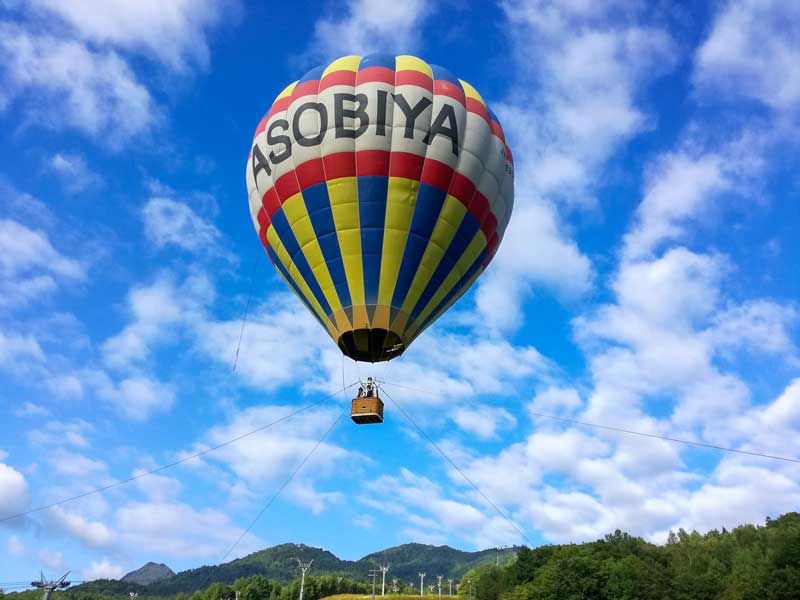In this vibrant photograph, a hot air balloon adorned with vertical blue and yellow stripes is captured in mid-ascent against a bright blue sky filled with fluffy white clouds. Horizontally across the balloon is a white banner bordered in red, bearing the text "ASOBIYA" in bold black letters. The balloon's woven brown basket, tethered to the ground with ropes, carries two individuals whose identities are indistinguishable due to the distance. Surrounding the scene, there are green trees, undulating hills, and several structures resembling power poles, adding to the picturesque landscape.